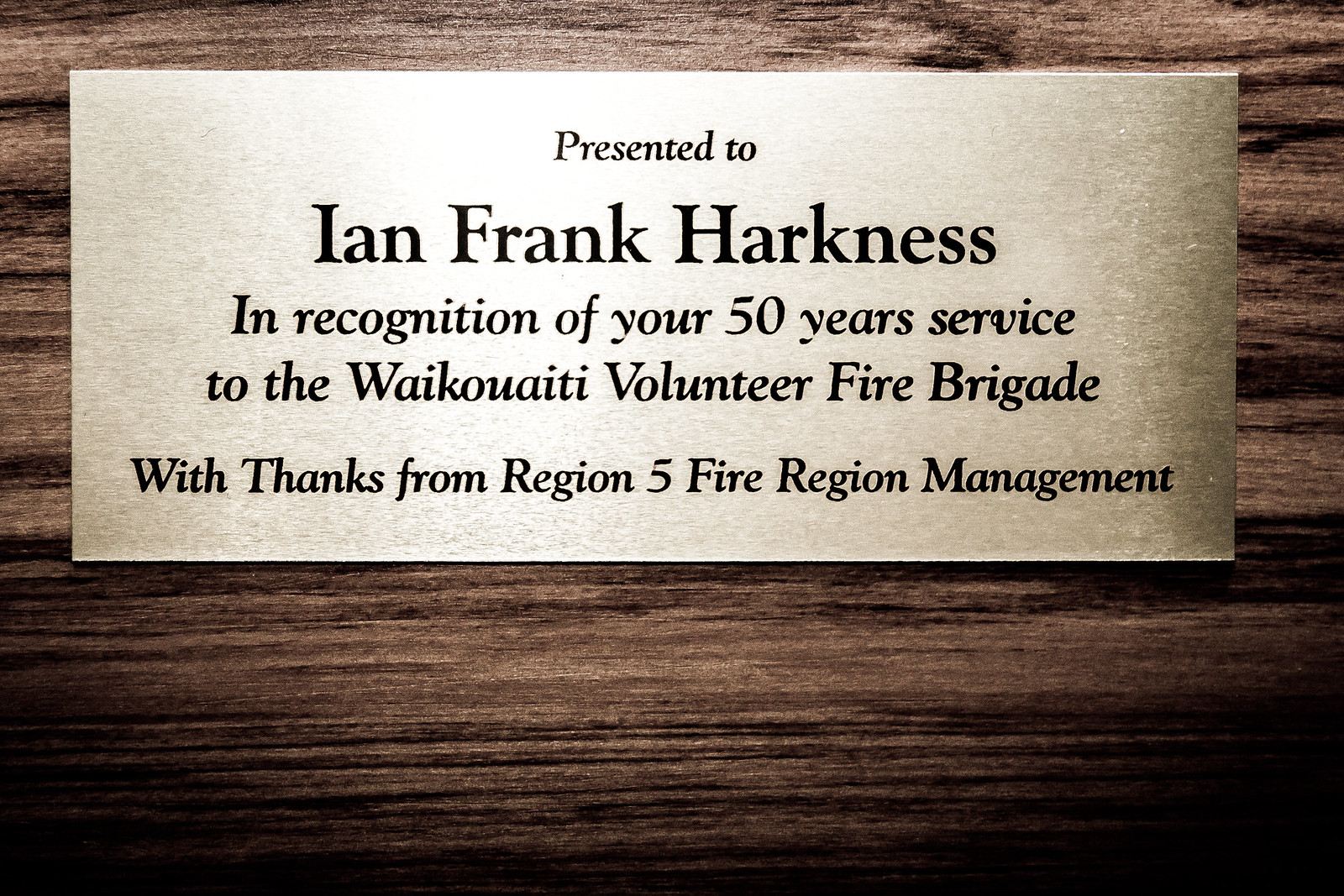This is a detailed photograph of a rectangular plaque placed on a dark wooden surface, possibly oak. The plaque features a silver nameplate with engraved black lettering. The text on the nameplate reads: "Presented to Ian Frank Harkness in recognition of your 50 years of service to the Waikuatiti Volunteer Fire Brigade, with thanks from Region 5 Fire Region Management." The light source gleams off the engraved letters, highlighting the formal tribute. The plaque itself is cream-colored, adding a refined contrast to its dark wooden background. The image provides an up-close, clear view of the lettering, capturing the essence of a well-deserved recognition award for long-term service in a Hawaiian fire brigade.